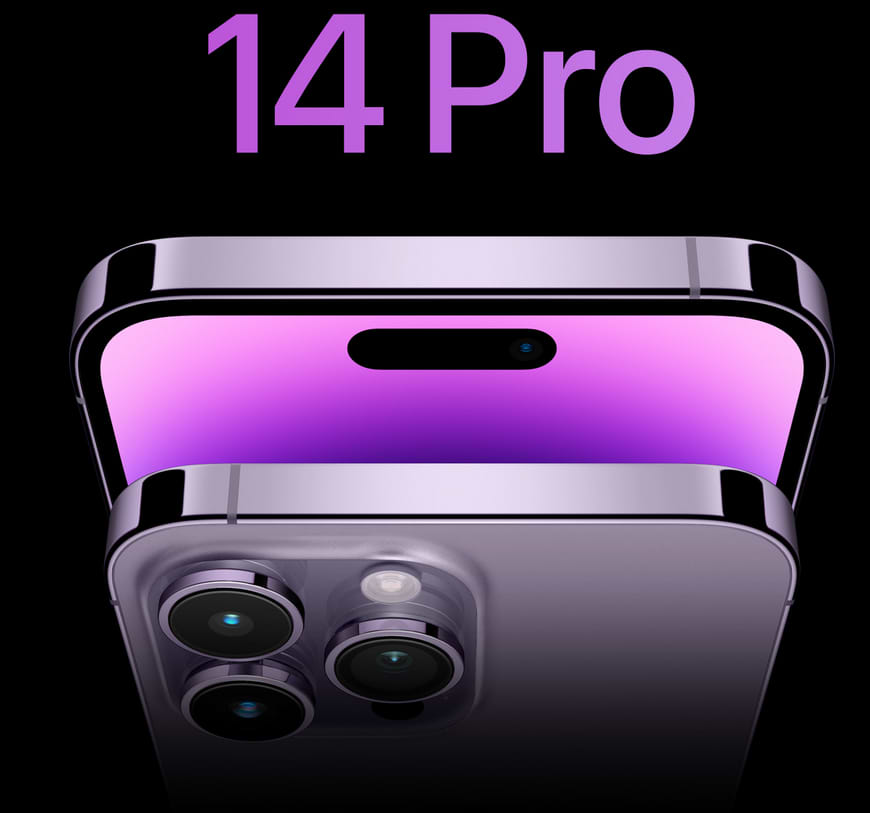The display ad showcases the Apple iPhone 14 Pro in a square format against a stark black background. Dominating the top of the ad, bold purple text prominently displays "14 Pro," immediately identifying the product being featured. 

Centrally placed beneath the text, the ad features a stylized composition highlighting two partial views of the iPhone 14 Pro. The upper image provides a glimpse of the phone’s front edge, showcasing a hint of the screen that gradients through various shades of purple and lavender. Below this, a second image offers a vantage point of the phone’s back, revealing its sleek silver finish. This angle focuses on an up-close view of the distinctive camera array featuring three cylindrical lenses arranged within a slightly raised, square-shaped module on the left side of the device.

The ad relies entirely on the iconic design and brand recognition of the Apple iPhone 14 Pro, with no additional text or elements crowding the visual presentation.